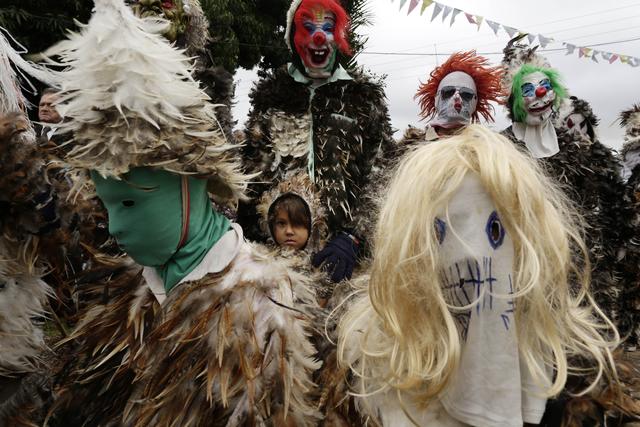The image depicts a lively scene from what appears to be a festival or parade, showcasing around ten individuals clad in an array of elaborate and eccentric costumes. Foremost, two figures stand out: the one on the left is almost entirely enveloped in fur except for a green stocking-like mask covering their head, with additional fur accessorized as a hat fastened under the chin. To their right is a figure donning a haunting mask resembling a ghost, featuring black eyes and crudely drawn teeth, complemented by an unkempt yellow wig. Between them, a child's face peeks out, encircled by a furry hat, appearing to stand in front of an adult, possibly a parent. The other participants in the background are similarly adorned in unsettling costumes, many featuring furry materials, masks resembling clowns or animals, and wigs of various vibrant colors such as red and orange, adding to the vivid tableau. The backdrop includes festive banners and bunting, enhancing the celebratory yet eerie atmosphere of the gathering.